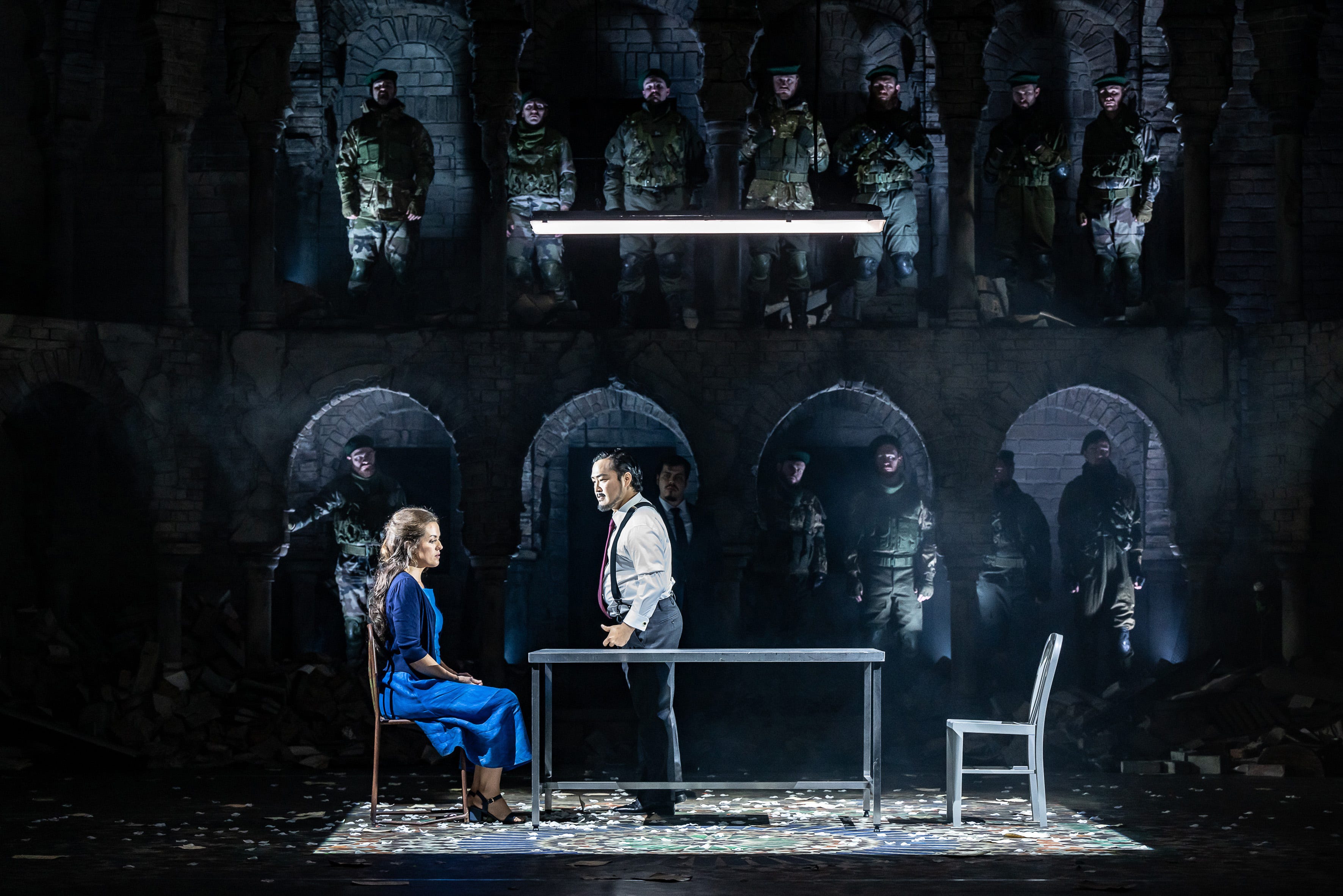The image captures a scene from a theatrical performance set in a two-story stage with a dark, rock-textured backdrop characterized by oval archways—four on the top level and four on the bottom. Within these archways, soldiers dressed in dark green military attire stand in shadow, their arms at their sides, creating an ominous and foreboding atmosphere. Their faces and forms are dimly illuminated, contributing to the menacing setting that resembles a villain's lair. 

At the center of this dramatic tableau, under a bright, focused light hanging above, a simple rectangular metal table rests on the stage. On one side of this table, an empty silver chair contrasts with a brown wooden chair occupied by a woman in a long, elbow-length blue dress and black sandals. She has long, light brown hair and is looking down, her hands resting in her lap, which underscores her solemn demeanor.

Facing her and standing slightly to the right, is an authoritative figure, possibly of Asian descent, dressed in dark gray pants, a white button-down shirt, black suspenders, and a red tie. His stern expression and posture, combined with his position over the table, suggest he is reprimanding or questioning her, adding to the tension and gravity of the scene.